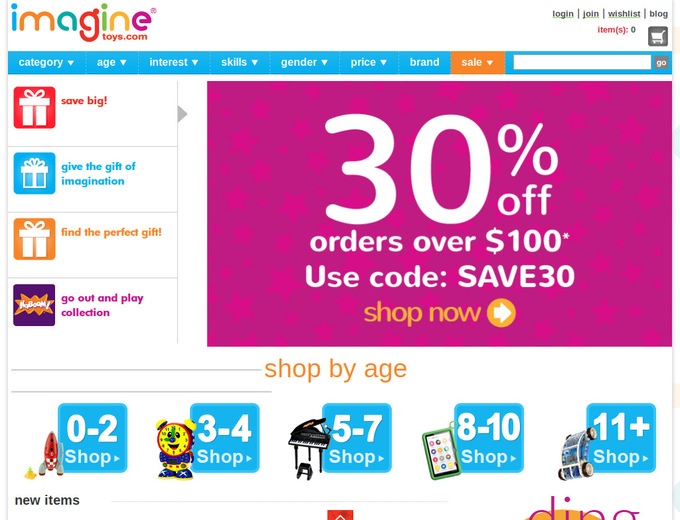**Description for imaginetoys.com Landing Page**

The **Imaginetoys.com** website features a clean and intuitive navigation bar across the top of the page. The navigation bar includes categories like **"Category," "Age," "Interest," "Skills," "Gender," "Price," "Brand," "Sale,"** and a **search bar** for easy browsing. Above this bar are options for **login, join, wishlist, blog, items (currently zero)**, and a **shopping cart icon.** The navigation bar and search criteria menu are highlighted in a bright blue color for easy visibility.

On the left-hand side of the page, promotional messages encourage visitors to **"Save Big," "Give the Gift of Imagination," "Find the Perfect Gift,"** and discover the **"Go Out and Play Collection."**

The primary image at the center of the screen features a vibrant **purple background adorned with pink stars.** The text on the image announces a special offer: **"30% off orders $100*"** with the code **"SAVE30."** The **"30% off"** text is predominantly styled in white font, while the **"SHOP NOW"** call-to-action button is highlighted in eye-catching orange, accompanied by a right-pointing arrow.

Below this promotional image, visitors can shop by age group, with options segmented into **ages 0-2, 3-4, 5-7, 8-10,** and **11+.** Each age group button is styled in blue with a white font and a right-pointing arrow, making it easy to navigate.

Further down, though partially cut off and unreadable, is a section labeled **"New Items."** The entire site maintains a crisp white background, ensuring that all categories and promotional elements stand out clearly.